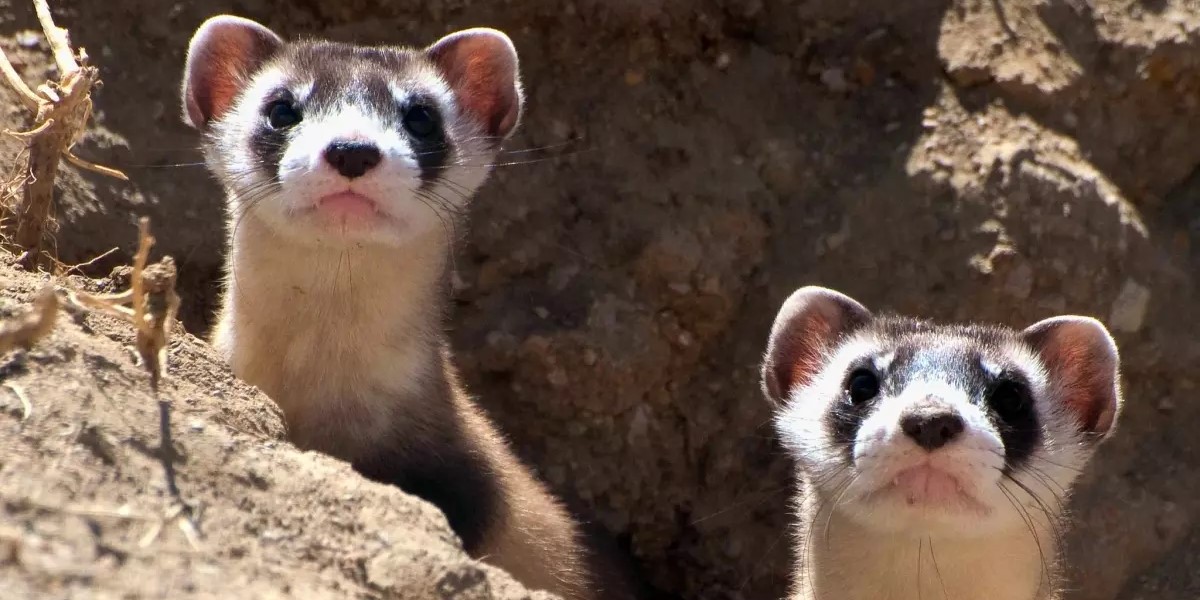This detailed photograph captures two prairie dogs peeking out from their burrow, which is partially underground. Their heads, adorned with short cat-like ears, are emerging from a dirt and rock substrate, surrounded by some dried, lifeless plants. The sunlight bathes their faces, emphasizing their distinct features: cute black noses, long black whiskers, and expressive eyes outlined with black fur. The prairie dog on the left is slightly more elevated, revealing more of its white neck that fades to brown, while the one on the right shows only the top of its head and neck. Both animals have pink lips and a mix of brown and white fur covering their bodies. The intricate detail in their whiskers and the subtle blend of their fur shades make them look adorably inquisitive as they gaze up at the camera, creating a captivating and intimate view of life in the wild.